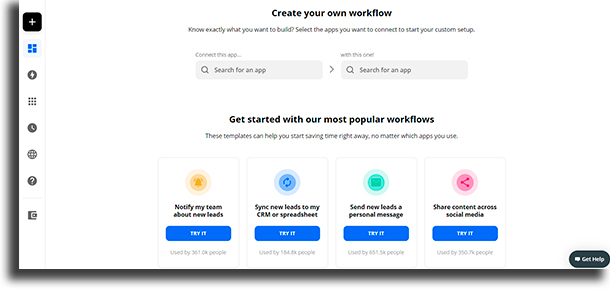Screenshot showcasing a workplace website interface for creating custom workflows. 

At the top, bold text reads "Create your own workflow," followed by a subheading that states, "Know exactly what you want to build. Select the apps you want to connect to start your custom setup." Directly below this, two adjacent search bars allow users to input and connect different applications, labeled "Connect this app" and "with this one."

Underneath, there's a section titled "Get started with our most popular workflows," accompanied by a note that says, "These templates can help you start saving time right away no matter which apps you use." 

This section is divided into four distinct, colorful boxes, each featuring unique symbols and text:
1. A yellow box with a bell icon, labeled "Notify my team about new leads."
2. A blue box with a refresh icon, labeled "Sync new leads to my CRM or spreadsheet."
3. A green box with a mail icon, labeled "Send new leads a personal message."
4. A red box with a share icon, labeled "Share content across social media."

Each box is visually designed to represent various workflow templates that can be customized to enhance productivity.